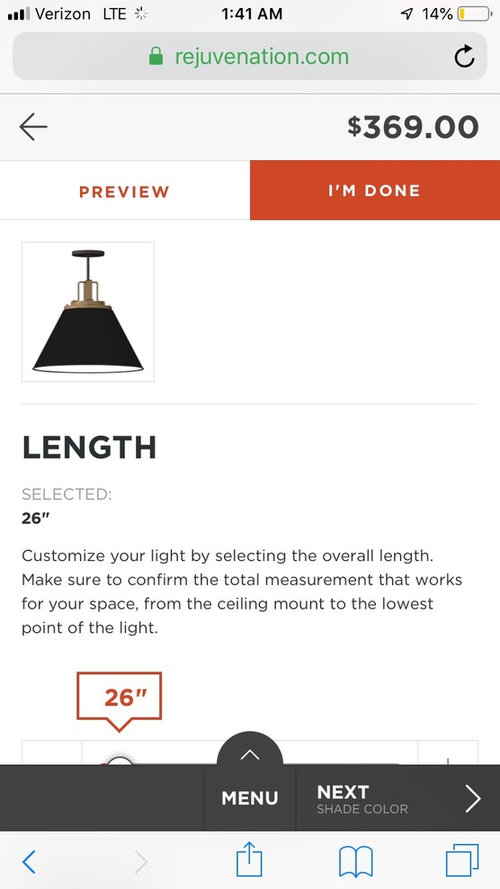This is a detailed screenshot of a smartphone display against an off-white background.

At the top-left corner, the screen displays a Wi-Fi signal icon with three out of four bars in black, indicating network strength. Next to it, the carrier name "Verizon LTE" is displayed in black text. Centrally placed in bold black letters, the time reads "1:41 AM." On the top-right corner, the battery icon shows only 14% charge left, with a yellow sliver indicating the remaining battery life.

Beneath this information sits a light gray navigation bar. A green lock icon signifies a secure connection, next to which the website "rejuvenation.com" is written in green text. A reload icon rests on the far right of this bar. 

Directly below, in a lighter gray section, is the price "$369" prominently displayed in bold, large black letters towards the right. Beneath this price, on the left, there is a whitish-colored button with red text that reads "Preview" and to its right, a red button with white text labeled "I'm done."

Under the "Preview" button is an image of a conical-shaped ceiling lamp, black with a white interior, hanging from the ceiling. Below the lamp image, informational text reads: "Length Selected is 26 inches. Customize your light by selecting the overall length. Make sure to confirm the total measurement that works for your space from the ceiling mount to the lowest point of light." Below this text, inside a box, the number "26 inches" is displayed in red.

Across the bottom of the screen is a black horizontal bar featuring a white arrow in a rounded center, pointing upwards, above the word "Menu" in bold white letters. To the right of "Menu," the word "Next" is written with a right-pointing white arrow next to it. At the very bottom-left, there is a blue back arrow. Under "Menu," a blue square with an upward-pointing arrow is displayed. Beneath "Next," an icon of an open blue book outline is present. On the far right, two overlapping blue squares are positioned, one atop the other.